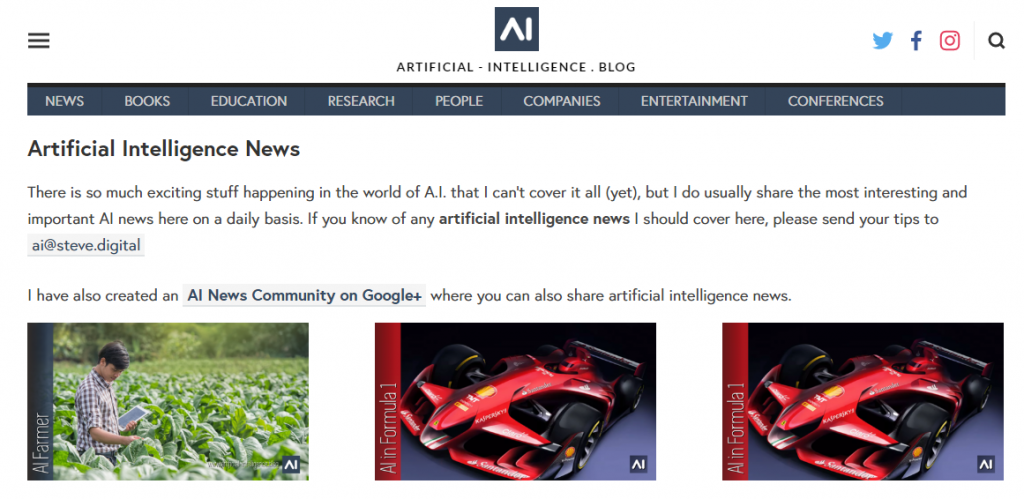A screenshot of an Artificial Intelligence blog. 

In the upper left-hand corner is the familiar three horizontal bars icon, indicating the menu. Centered on the screen is a greenish-gray block featuring the white silhouette of an AI figure, representing the website's logo. Below this logo, also center-justified, is the text "Artificial Intelligence Blog." 

In the upper right-hand corner are icons for Twitter, Facebook, Instagram, and a magnifying glass for search. Beneath the blog title, a gray navigation bar spans the screen, containing white font menu items from left to right: News, Books, Education, Research, People, Companies, Entertainment, and Conferences. 

Dominating the page is the main article titled "Artificial Intelligence News." At the bottom of the screen, three blocks of pictures are displayed, hinting at additional content or related articles.